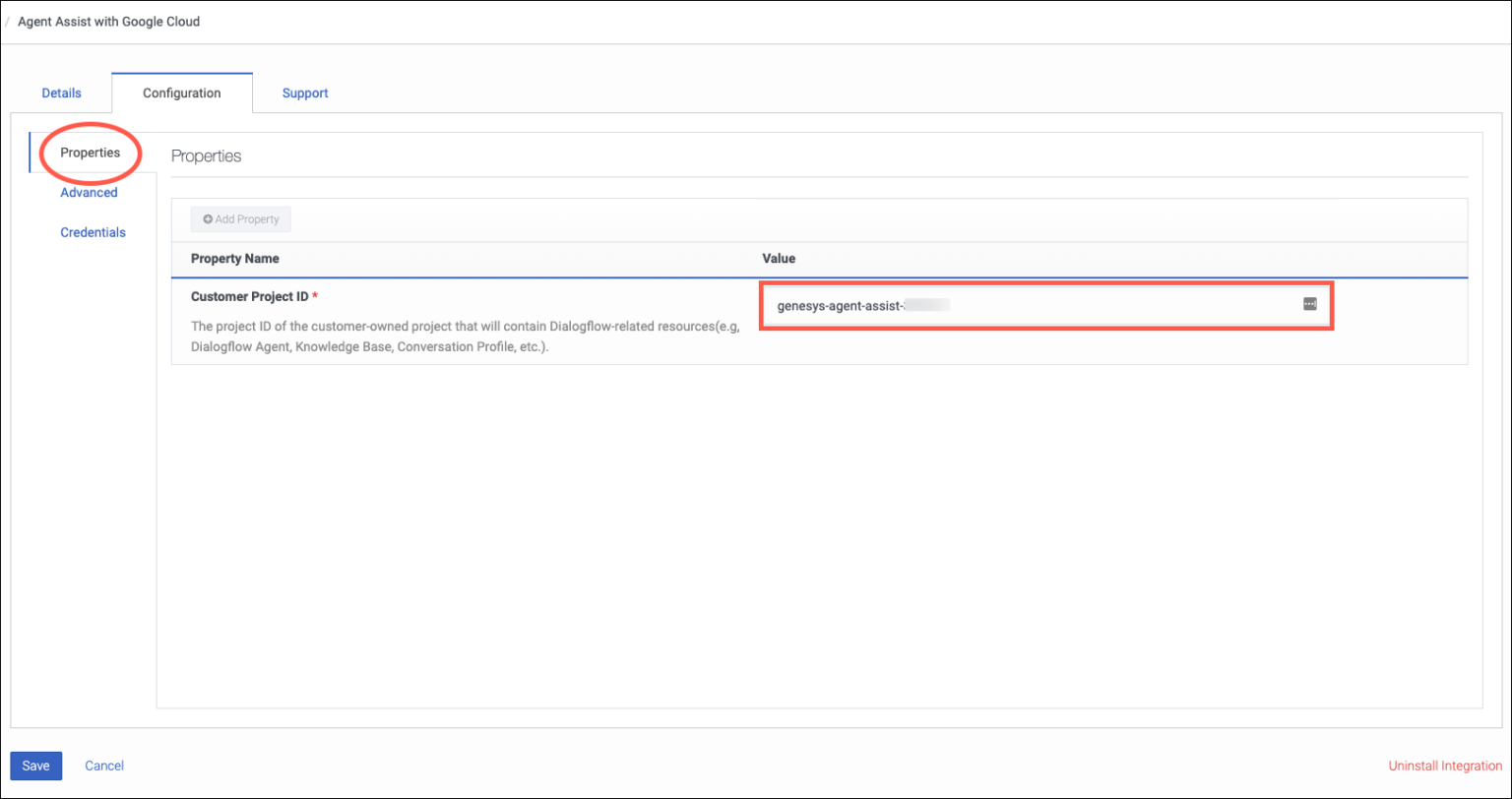This image showcases a detailed configuration screen for "Agent Assist" with Google Cloud, set against a white background. In the top left corner, the header "Agent Assist with Google Cloud" is prominently displayed in black text. 

Below the header, three primary sections are labeled: "Details" in blue, "Configuration" in black, and "Support" in blue. Underneath these sections, there is a subheading "Properties" in black font, encircled by a bold red circle. Further down, "Advanced" and "Credentials" are labeled in blue text.

To the right of the circled "Properties," the word "Properties" appears once more. Below, there is a search or text entry box with the prompt "Add Property.", followed by the label "Property Name." Further beneath, the term "Customer Project ID" is indicated, marked with a red asterisk, signaling a required field.

The section explains that this ID pertains to the customer's project that will house Dialogflow-related resources, such as the Dialogflow Agent, Knowledge Base, and Conversation Profile.

Adjacent to this explanation, a white rectangle bordered in red displays the text "Genesis Agent Assist." At the bottom of the image, two action buttons are present: a blue rectangle labeled "Save" on the left, and the word "Cancel" in blueprint to its right.